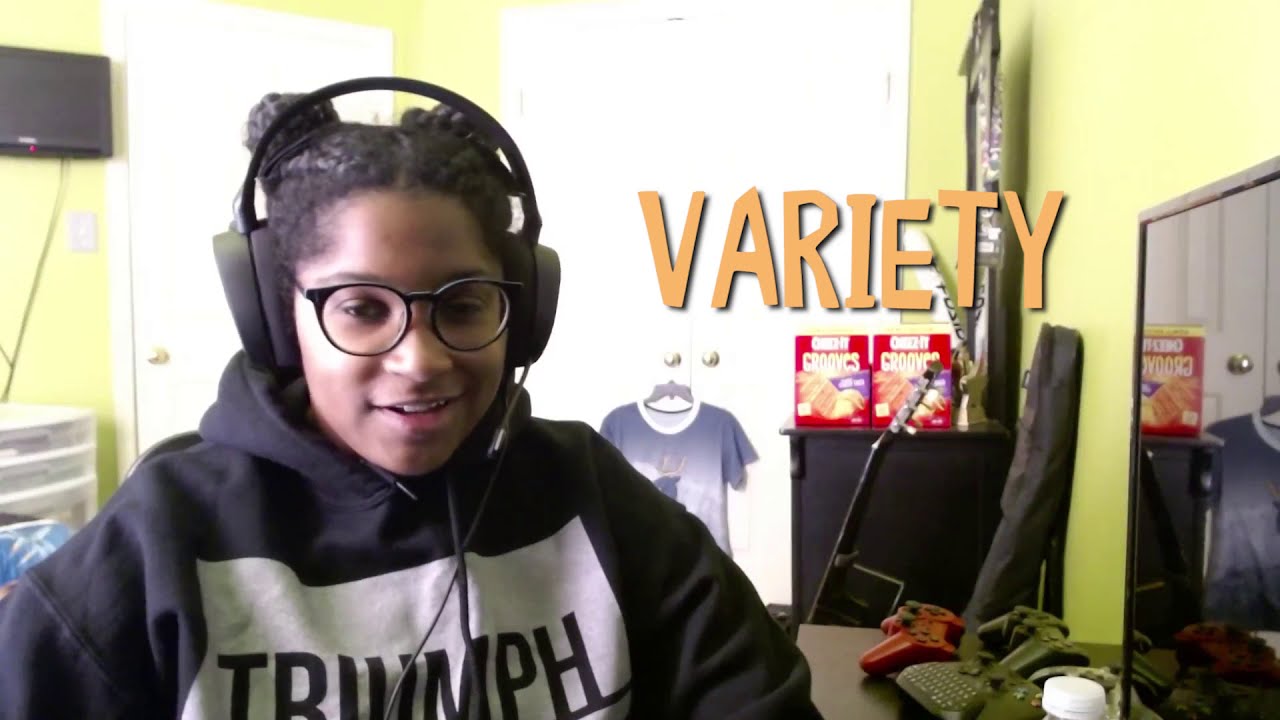The image, taken indoors in a brightly lit room with walls painted a light green color, features a girl sitting centrally, likely a gamer. She sports headphones with a microphone, sunglasses, and her hair styled in two buns. She wears glasses in some accounts and a black hoodie with a white banner across the front bearing the word "TRIUMPH" in black letters. 

Directly behind her, there's a white closet, flanked to the left by a white door and a white drawer tote above which a TV is mounted on the wall with visible cords. The phrase "VARIETY" in bold, orange capital letters is prominently displayed in the middle of the picture near the girl. To the right, there's a table holding remote controls and two boxes of Cheez-Its. A dresser is visible with a mirror reflecting a portion of the scene, and nearby, a red game controller and other items including what appears to be a guitar case and potentially other miscellaneous items like a gray object and a greenish item.